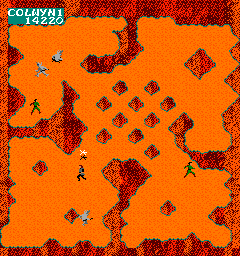In the year 14220, an expanse dominated by vivid hues of orange and red stretches out in all directions. The ground is primarily an intense orange, speckled with red dots that add depth and shading, creating a textured surface. Scattered across this vibrant landscape are patterns that resemble rocks. 

In the top left corner of the image, a bird is perched, intently observing a human figure below. This human, clad in a distinctive green shirt, stands out amid the fiery background. At the very bottom of the image, shades of gray blend with the scene, contrasting with the surrounding colors.

Additionally, a striking black and white starfish is visible, adding an element of marine life to the tableau. On the extreme right, another figure can be seen walking, characterized by their green shirt, dark belt and shoes, and a prominently styled pompadour haircut. Notably, the area appears confined, with no discernible entrances or exits, lending an air of isolation to the scene.